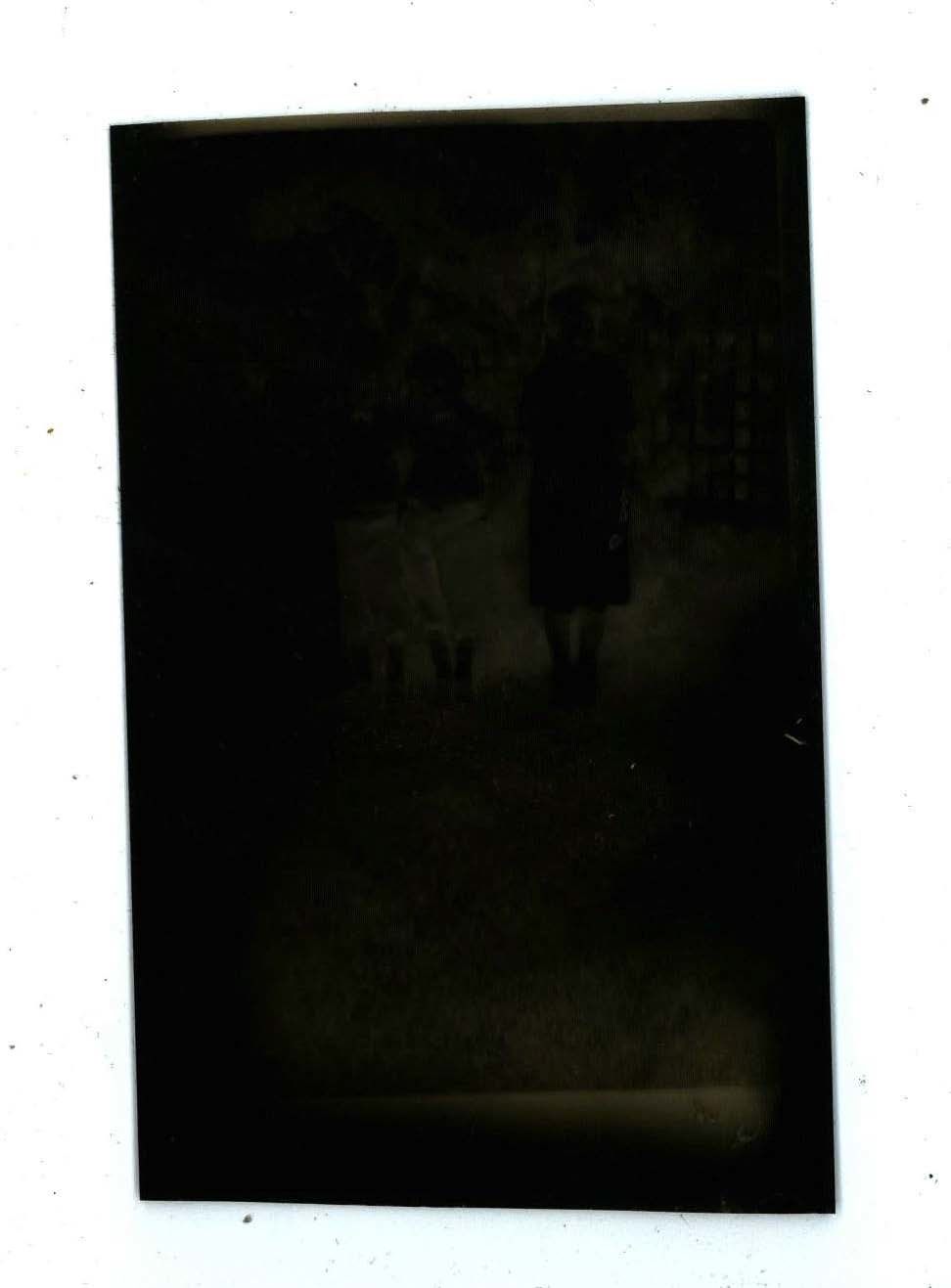In this dimly lit photograph, three small figures can be discerned from the shadows, possibly children due to their size. The image appears to have been taken outdoors, as suggested by patches of green grass and faint sunlight illuminating parts of the scene. At the forefront, a young girl stands tallest among the group, dressed in a knee-length dress. Flanking her are two young boys, each dressed in light-colored pants that reach just above their ankles and darker, short-sleeved tops. Behind them, a fence framed by lush greenery can be indistinctly seen, adding to the outdoor setting's ambiance.